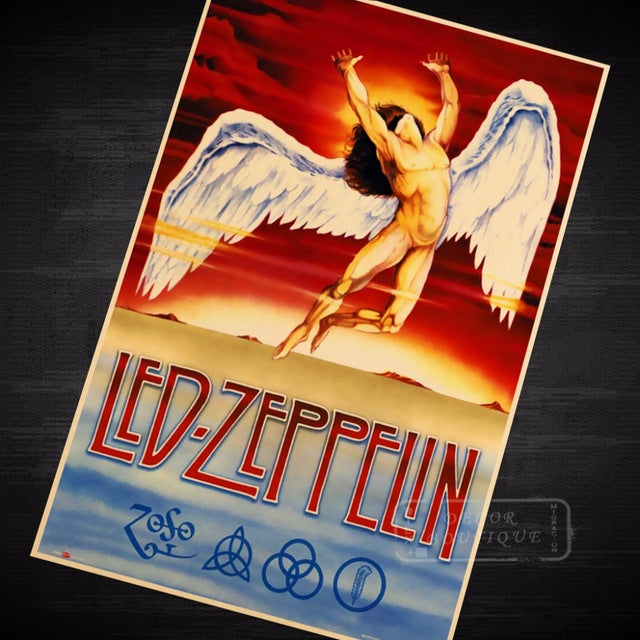The image depicts a booklet or insert related to Led Zeppelin, often mistaken for the album "Led Zeppelin III." The booklet features a striking design with a red sky and a yellow sun in the background. Dominating the foreground is a muscular, nude man with long brown hair and large white wings, reminiscent of an angel. This figure appears to be soaring, with his arms stretched upwards. The booklet's design includes a diagonal layout, placing it at an angle on a black background, making the top left and bottom right corners cut off. In red typeface, "Led Zeppelin" is emblazoned across the bottom of the image. Below this, four symbols are displayed: the first resembles the Olympic rings, and the remaining three are distinctive emblems often associated with the band. The overall color scheme transitions from a red sky to cream and blue tones at the bottom, creating a dynamic and visually engaging presentation.